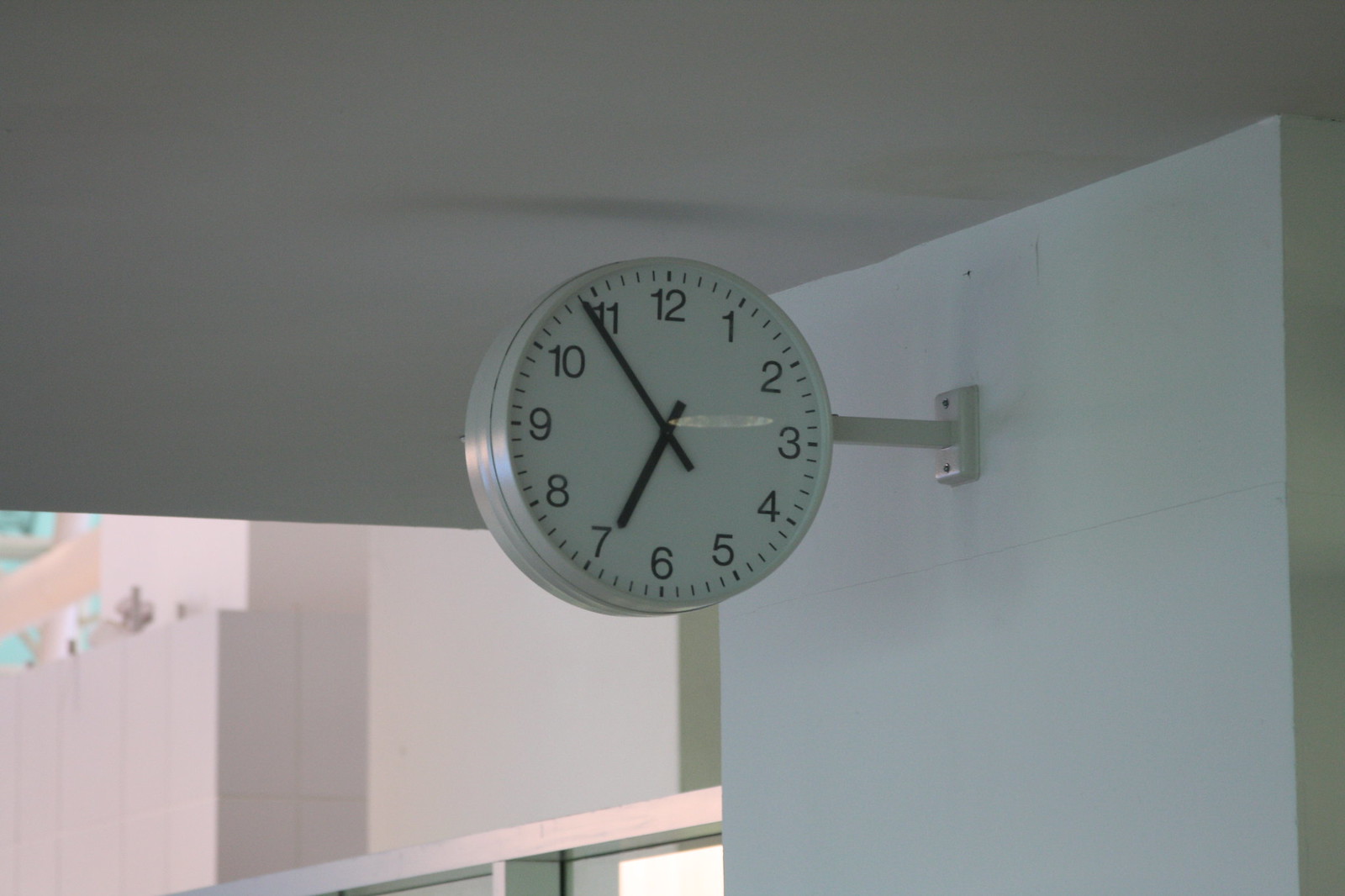This photograph features a uniquely mounted clock as its focal point. The clock, circular in shape, prominently displays a minimalist design with a black dowel and a sleek silver ring encircling it. Unlike conventional wall clocks, this one is affixed to a white brick wall via a sturdy metal pole extending from its side, providing an unconventional, off-the-wall appearance. The clock reads approximately six minutes to seven, and despite the dowel obstructing a clear view of the am/pm indicator, the evident sunlight suggests it is likely 7 a.m. Above the clock, a white ceiling transitions into a background composed of more white brick and tile, contributing to the overall bright and clean aesthetic. Notably, the background possesses an unusual, almost digitally-rendered quality, hinting at a potential AI or computer-generated origin.